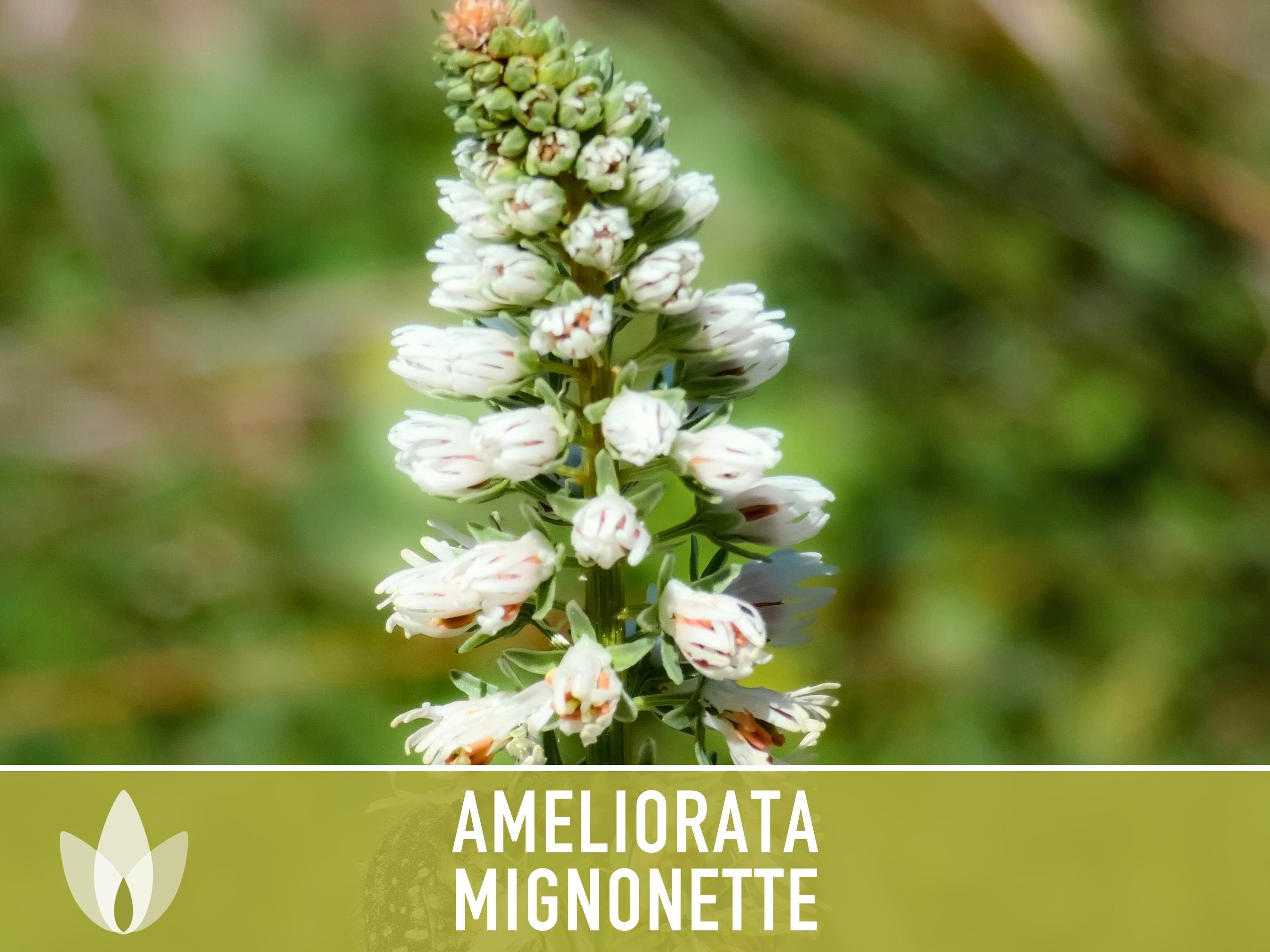The photograph depicts a tall, elegant flower known as Mignonette Ameliorata, prominently displayed in the center of the image. The flower is characterized by numerous white buds, interspersed with some green ones that have not yet opened. As you move down the plant, you can observe the progression of the buds opening, with those near the bottom fully in bloom, revealing silky, soft white petals. The background is intentionally blurred and features shades of green and a hint of pink, making the plant stand out sharply. Below the flower, there is a caption that reads "Emily Arada Mignonette," written in white on a lighter green-yellowish background, accompanied by a small logo to the left of the text. The image, possibly a framed picture or postcard, captures the intricate and delicately beautiful details of the flower, which is known for its use in floral bouquets and its violet-like fragrance.